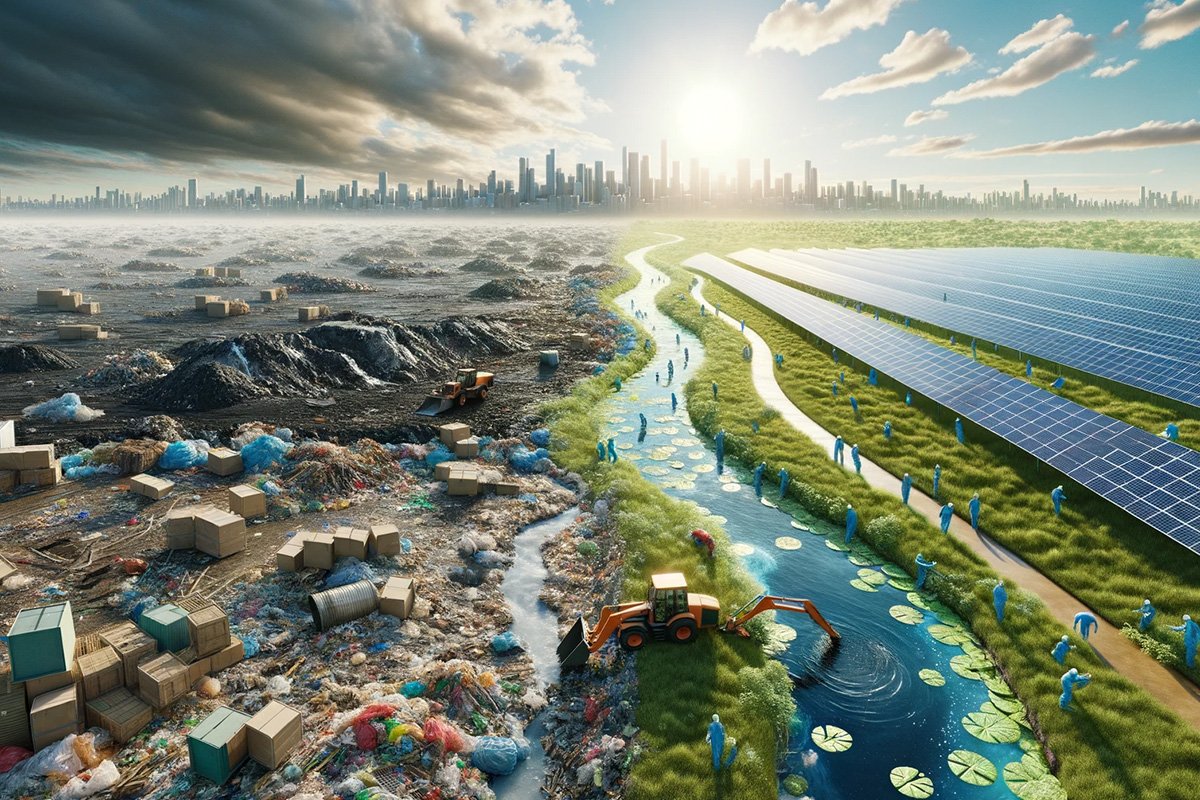The image, appearing to be computer-generated or a drawing, intricately depicts a stark transition between two contrasting environments. In the foreground, there is a wasteland filled with industrial garbage, including mounds of rocks, plastic, and barrels, all amidst a polluted waterway. A builder or tractor is actively dredging through the garbage and cleaning the river, while several people in blue hazmat suits are seen working and stretching into the distance. On the left side of the foreground, large piles of gray dirt and cardboard boxes dominate the scene. As your eyes move rightward from the center, the landscape becomes more lush with greenery and features a walkway leading towards expansive rows of solar panels that stretch into the horizon. The right fork of the waterway is adorned with large lily pads, contrasting with the polluted section. In the far distance, an urban skyline of gray skyscrapers looms under a partially stormy sky, with dark clouds on the sides and a bright sun breaking through in the middle, symbolizing a transition from pollution and waste to renewable energy and cleaner environments.